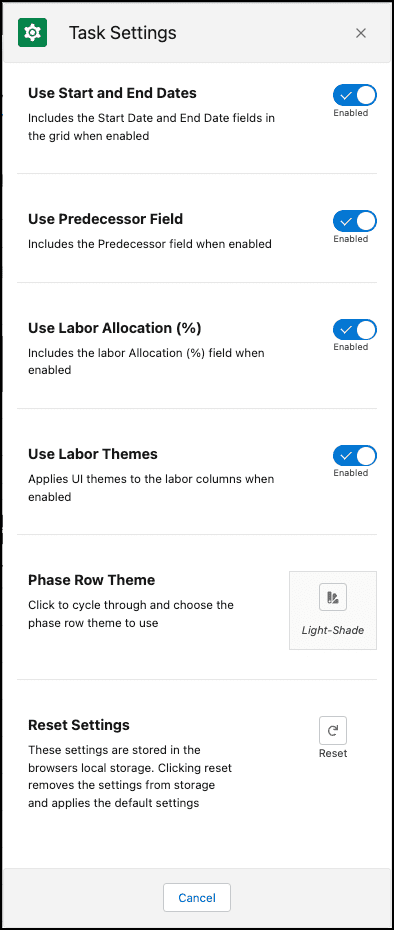A vertically rectangular image appears to be a screenshot from a cell phone, bordered by a thin black line. Positioned at the top left corner is a settings icon on a green background, with the text "Task Settings" to its right. Over in the upper right corner, there's an 'X' icon to close the window.

Beneath these elements, a list of settings is displayed, with the first four options featuring toggle switches on the right side, all of which are enabled. These options are:

1. **Use Start and End Dates**: This option includes the start date and end date fields in the grid when enabled.
2. **Use Predecessor Field**: This option includes the predecessor field when enabled.
3. **Use Labor Allocation Percentage**: This option includes the labor allocation percentage field when enabled.
4. **Use Labor Themes**: This option applies UI themes to the labor columns when enabled.

Following these toggles is the "Phase Row Theme" option, which invites the user to "Click to cycle through and choose the phase row theme to use." To the right of this instruction, a box labeled "Light Shade" is present.

At the bottom of the settings list, there is a "Reset Settings" option accompanied by a reset button on its right side. Centrally positioned at the very bottom of the image is a "Cancel" button.